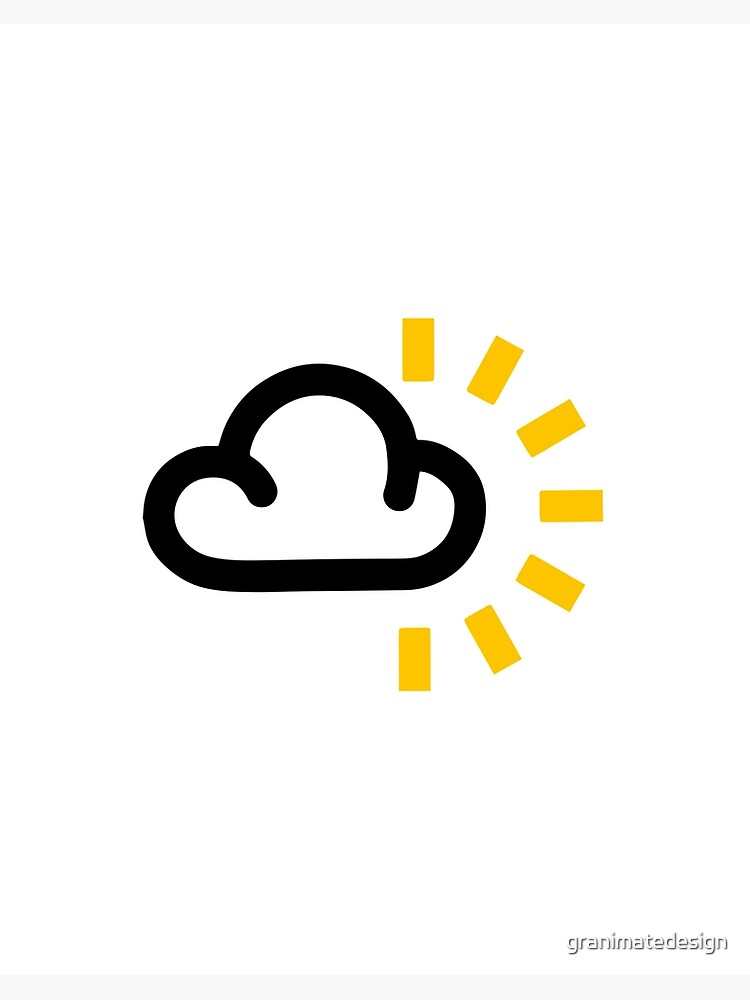The image features a simple, almost icon-like graphic, set against a white background. At the center is a stylized, puffy cloud, outlined in bold black with a white interior. On the right side of the cloud, eight equally-sized, yellow rectangles emanate in a semi-circular arrangement, giving the impression of sun rays peeking out from behind the cloud. The overall effect is a visual representation of partly cloudy or mostly sunny weather. Below the image, the text "granimate design" is written in a whitish-gray font. The design blends elements of graphic art and clip art, potentially serving as a symbol in news graphics or weather illustrations.